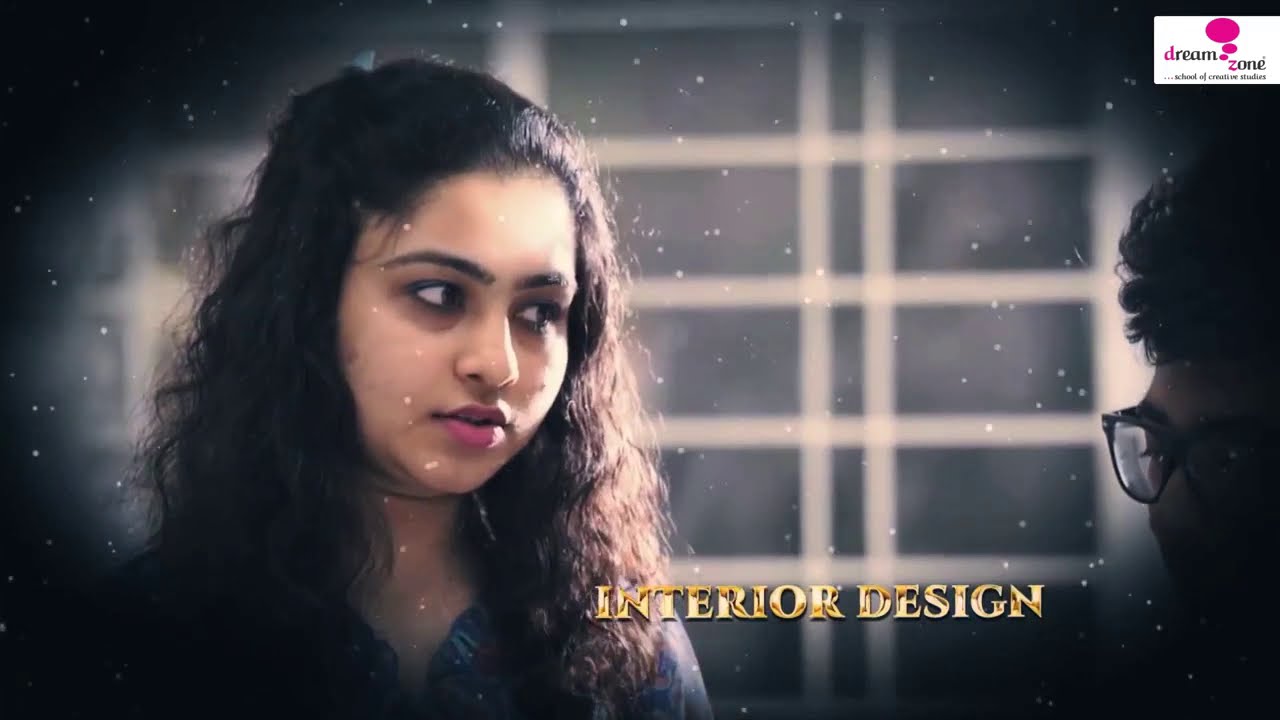The image appears to be a promotional ad or a screenshot featuring a young woman on the left side, who is in her 20s with long, flowing curly dark hair, dark eyebrows, dark eyes, and pink lipstick. She is wearing a purple top and has an open mouth, suggesting she is speaking to someone. On the right side of the image, there is a young man with thick, curly brown hair and black glasses, but his features are partly obscured by shadows and a black fading border. The background includes a doorway, creating a somewhat indistinct scenery. Overlaid on the bottom of the image in golden capital letters is the phrase "INTERIOR DESIGN." In the top right corner, there's a watermark/logo in a white box with pink and black text that reads "Dream Zone School of Creative Studies," accented with pink circles. The overall tone of the image is somewhat dark, especially around the edges.